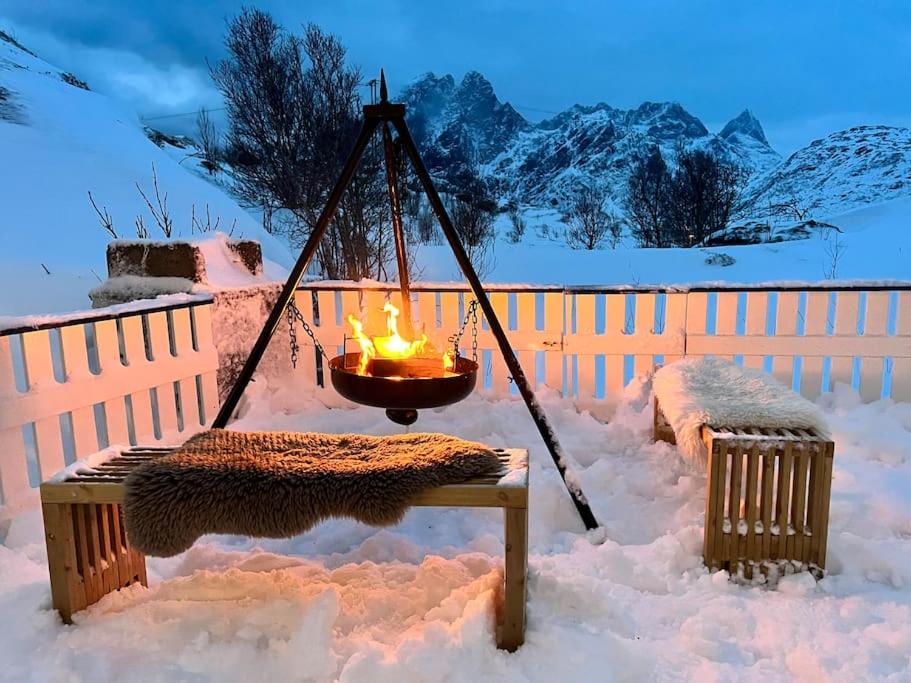In this cozy winter scene, a snowy backyard is nestled within a picturesque mountainous landscape. Snow-capped peaks and bare trees frame the background, while a gray, cloudy sky hints at evening approaching. The fenced-in yard is bordered by a white picket fence and blanketed in several inches of snow, disturbed enough to suggest frequent gatherings. At its center stands a black, cast-iron fire pit, suspended by a triangular stand and emitting a warm, inviting glow. Flanking the fire pit are two wooden benches, each draped with thick fur blankets, one brown and one white, enhancing the overall coziness. Despite the absence of people or animals, the setup exudes a sense of warmth and comfort, making this backyard a perfect, serene retreat amidst the snowy wilderness.